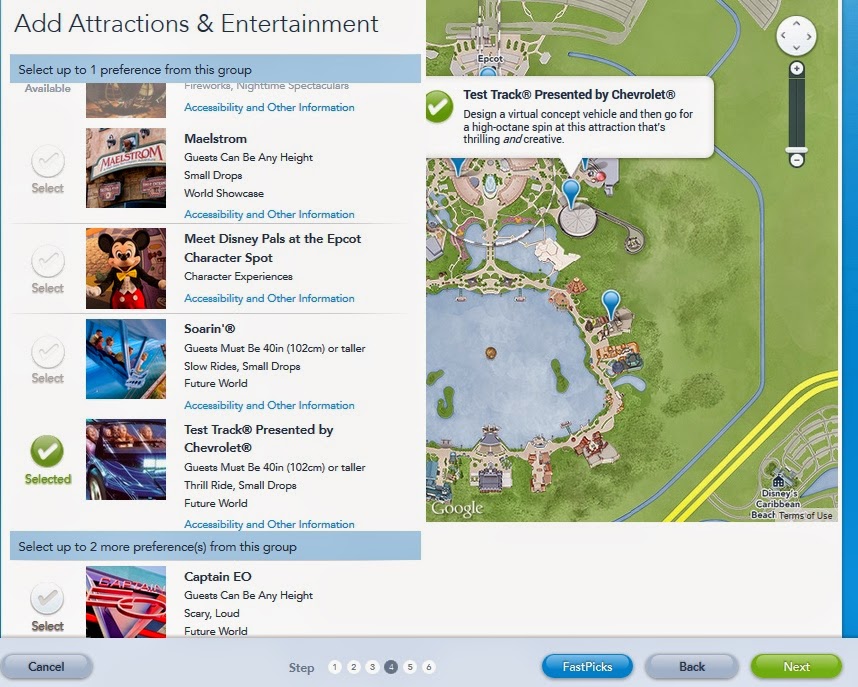This detailed caption describes an image from a Disney theme park attraction selection interface:

"The image displays an interface from a Disney theme park, specifically Epcot. At the top, there is a header titled 'Add Attraction Entertainment,' followed by a blue subheader prompting users to 'Select One Preference.' Below this header, there are selectable options listed, with the only available option being highlighted in green with a check mark next to it.

The content beneath the header begins with a section on accessibility. The first selection is partially cut off, but to its right reads 'Accessibility and Other Information' in blue text. Below this, there's a note indicating that the attraction is called 'Meet strum,' and guests can be of any height. It also mentions 'small drops' and the 'World Showcase.' Continuing with accessibility and additional details in blue, the next listing shows 'Meet Disney Pals at Epcot Character Spots.' This section includes a picture of Mickey Mouse sporting his classic tuxedo, yellow bowtie, and red pants.

Following that, there's information about the 'Soarin'' attraction, which includes height requirements. The subsequent attraction listed is the 'Test Track presented by Chevrolet,' which is marked with a green check.

Further down, there is another blue box with the prompt 'Select up to Two More Preferences from This Group,' which currently has no marked selections. Under this prompt, there is an option labeled 'Captain EO.'

To the right of the selections, there is an image of the Epcot map, complete with a legend indicating directions (North, South, East, West), and zoom in and out buttons. The map highlights the exact location of the selected 'Test Track' attraction with a pin, showing its precise position within Epcot Center."